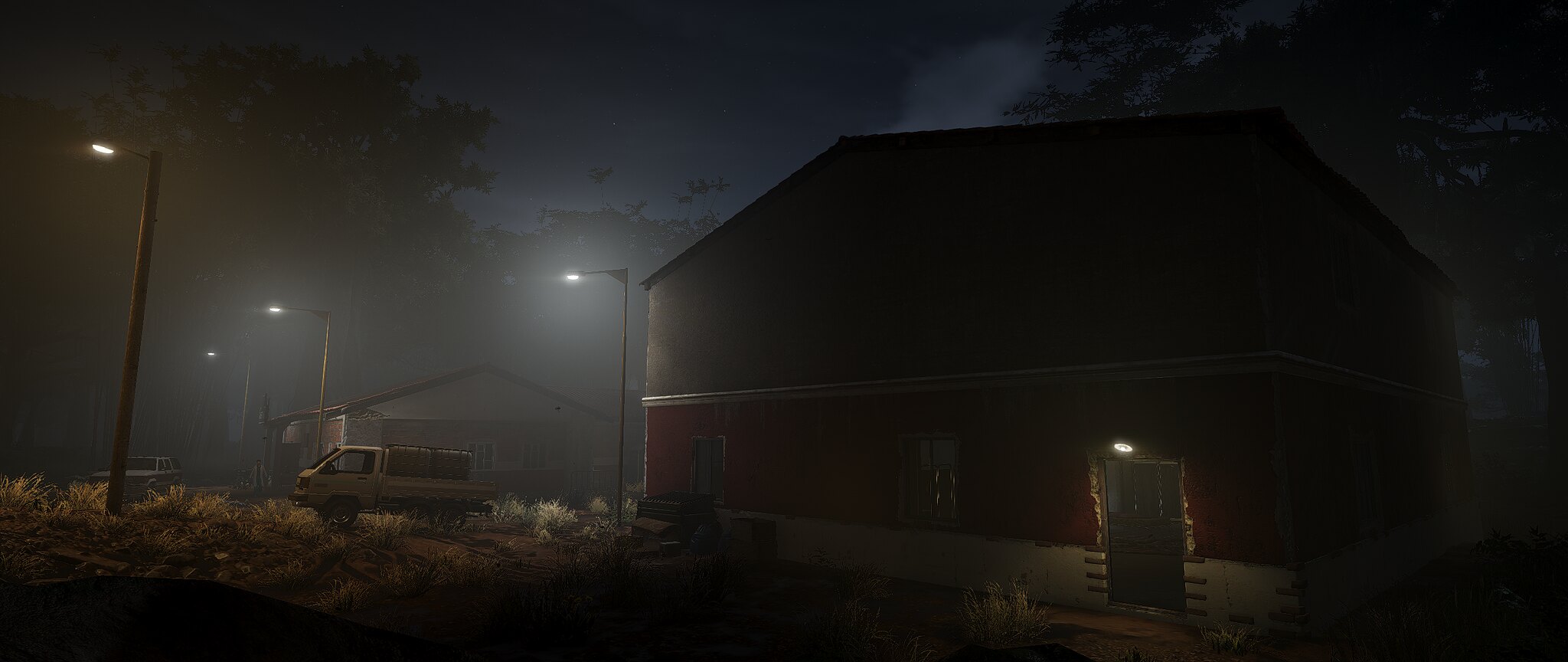This nighttime still image from my video game depicts a two-story building featuring a distinct color palette and architectural details. The lower section of the building is adorned with red and white hues, transitioning from a white base to a deep red facade. The upper section contrasts sharply with its dark charcoal-gray color. A door, accented by a hanging light directly above it, is situated on the far right side of the building. The structure includes two windows: one centrally located and another positioned on the far left.

To the left of the building, a small beige truck is parked, adding to the scene's realism. Four light poles are scattered around the property, providing illumination. A white garage with a black roof and double doors is visible in the distance to the left of the main building. Additionally, multiple tree silhouettes frame the scene, enhancing the atmospheric setting.